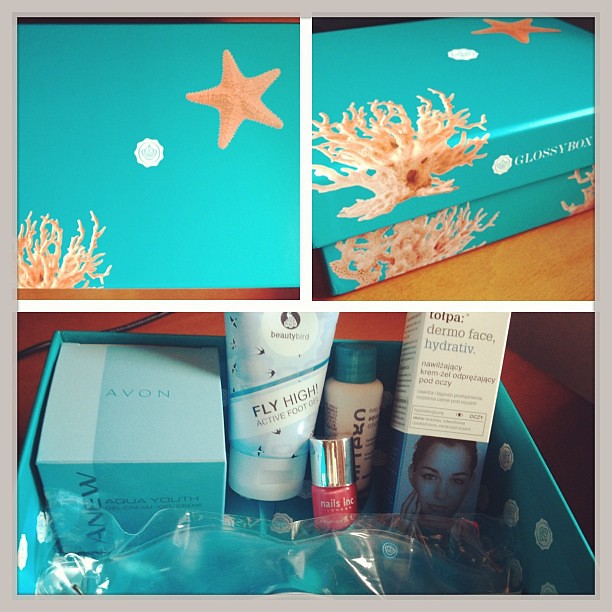This collage consists of three images showcasing a turquoise (Tiffany blue) box adorned with a beige-golden starfish on the right edge, coral on the bottom left, and a white logo that reads 'Glossy Box'. 

The first image displays the top of the box on a wood-grained surface, highlighting the elegant sea-themed design. The second image captures the box from a side angle, extending the coral and featuring the white 'Glossy Box' logo prominently. The third image reveals the box's contents: a large Avon Anu box, a Fly High Active Foot Cream tube, a dermo face hydra-tive box with a woman’s face illustration, a bottle of pink nail polish, another unidentified medium-sized bottle, and what appears to be a gel face or eye mask. The interior of the box is also turquoise with white decorations, aligning perfectly with the exterior theme. The entire collage is framed by a pale gray border, adding a touch of sophistication to the presentation.